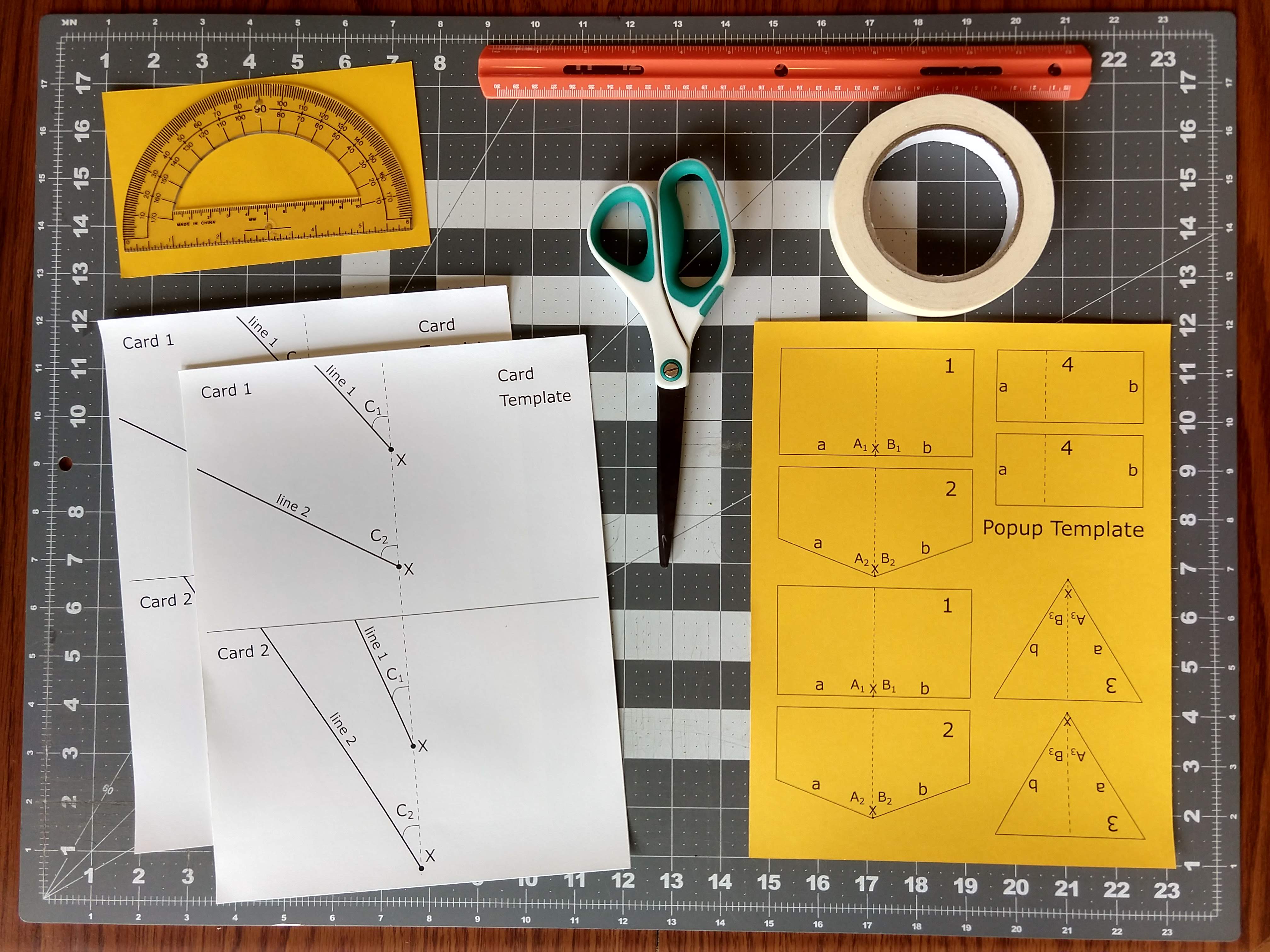This is a detailed photograph of a workspace likely used for precision tasks such as crafting or small-scale construction. The scene is set on a rich, brown wooden desk, and is dominated by a large measuring mat that features an array of geometric shapes, numbers, rulers along its edges, and grids for accurate measurements. At the top center of the image, there's an orange ruler lying horizontally with a roll of masking tape just below it. To the left of the masking tape, a pair of scissors with green and white handles is prominently placed. Moving further left, there is a notable yellow, possibly orange, piece of paper partially covered by a circular measuring tool. Nearby, two white pieces of paper labeled "card template" display drawings of lines and other shapes. Beneath these templates is another sheet marked "pop-up template," featuring a detailed layout with numbers and letters indicating folds and cut-outs. This mixture of tools and templates strongly suggests that the desk is prepared for intricate project work involving precise measurements and cuts.